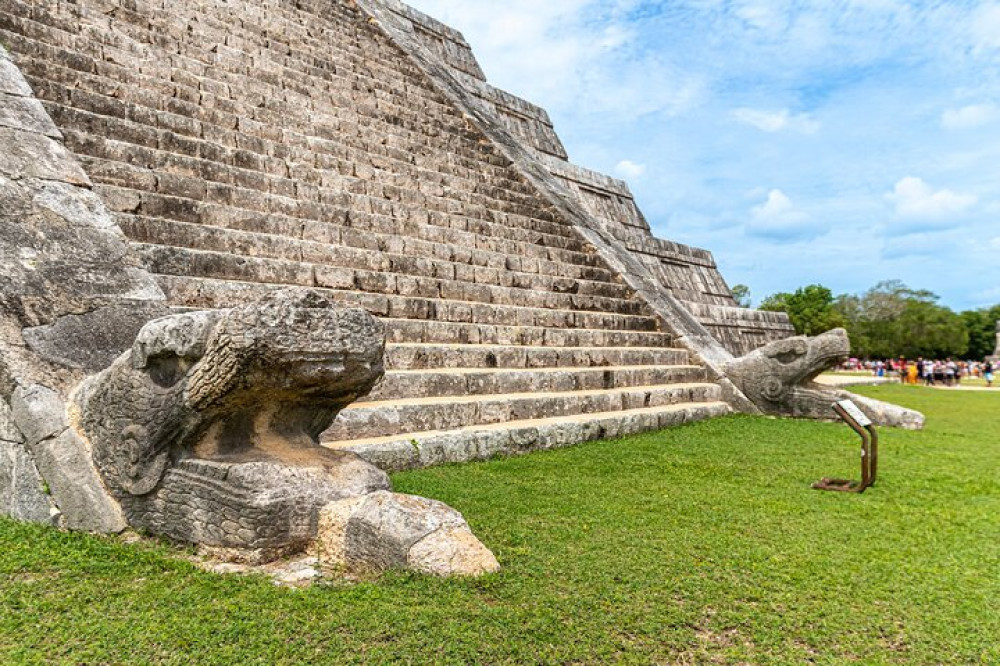This color photograph captures the majestic base of a historic Mayan temple, likely Chichen Itza, known for its distinctive pyramid structure with rustic stone steps ascending into a mostly clear blue sky. Dominating the left side of the image, the temple's staircase is flanked by intricately carved serpent heads, likely representing Quetzalcoatl, the feathered serpent deity revered in Mayan culture. At the bottom right, a well-manicured grassy area adds a vibrant touch to the scene, leading up to a prominent white informational sign mounted on a brown base, although the text is not legible due to the angle. Scattered in the background along pathways, small groups of people can be seen, evoking the sense of a dynamic yet historical setting. The overall atmosphere suggests it was taken in the afternoon, with the sunlight casting a gentle illumination over the ancient stone textures.